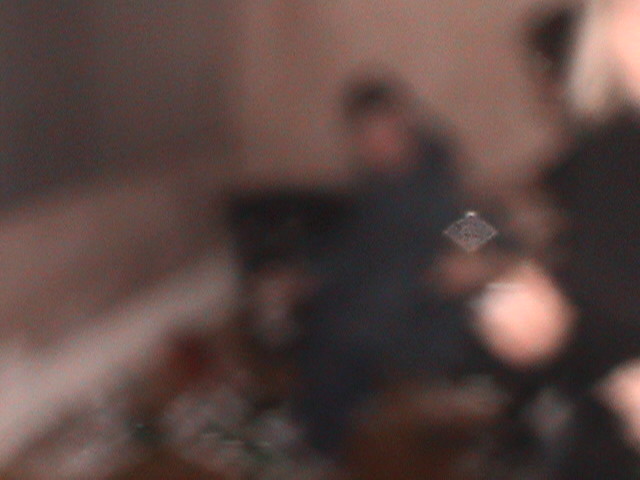The image is a very blurry photo that seems to depict two people. One figure sits more centrally, dressed in what appears to be a gray or blue hoodie, possibly dark blonde or brown-haired, with skin darker than a Caucasian. The second person, positioned towards the extreme right and partially cut out of the frame, wears a black hat and is dressed in black, with black hair. Both individuals seem to be seated, potentially on a chair or sofa, with some suggesting they might be looking at each other. Underneath them, there's a reddish or brownish rug or carpet, and the surrounding area indicates a dimly lit indoor setting, likely with a white or grey wall in the background, maybe suggesting a blue tint on the left side. A glaring bright white spot and a peculiar opaque diamond-shaped object appear between the two figures, possibly resulting from exposure issues, such as interference from a flash or other image artefacts. The photo overall is heavily glared, almost giving the impression of an overexposed old Polaroid image, which adds to its eerie and ambiguous feel.